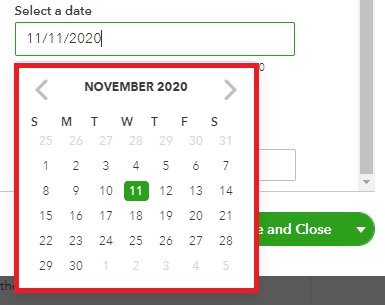The image showcases a close-up screenshot of a digital date selection interface. In the upper left-hand corner, the text "Selected Date" is displayed in small, black font with a capital "S" in "Selected". Below this label, there is a white text input box bordered in green, containing the date "11-11-2020" with the cursor positioned at the end of the date. Beneath the input box, a pop-up calendar is visible, set to November 2020. The calendar highlights November 11th, with left and right arrows flanking the month and year, allowing navigation to previous and next months. The bottom section of the image features a black bar, possibly part of the application's background, and to the right side, a green "Save and Close" button is visible.